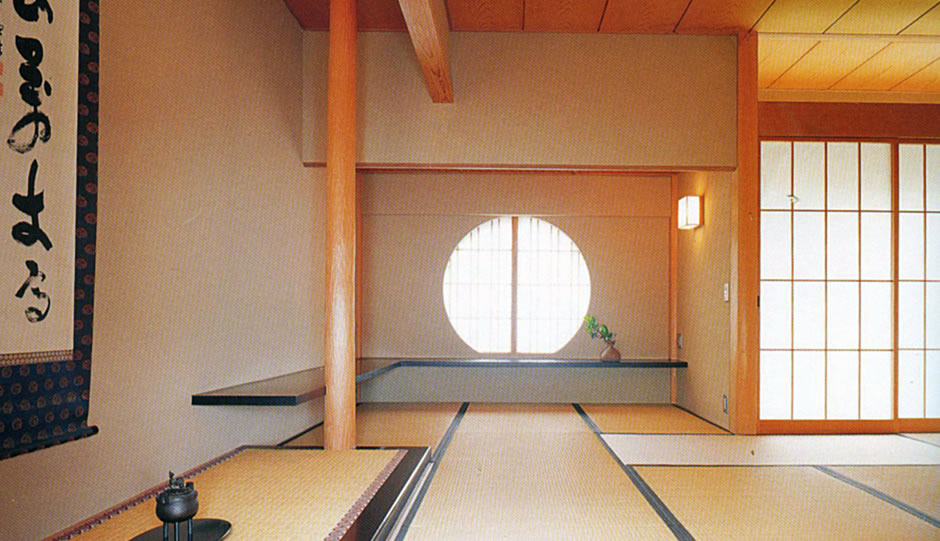This photograph depicts a serene, spacious room with traditional Asian design elements, possibly inspired by Japanese aesthetics. The room features a wooden or straw floor with dark accents, creating a warm, earthy atmosphere. Dominating the left side, a vertically hung scroll with black characters on a white background, bordered in blue and gold, adds an elegant touch to the plain walls. A low table, positioned near the floor, holds a small black pot with three legs, suggesting simplicity and functionality.

At the center of the room stands a sturdy wooden column, supporting the ceiling's wood panels, which are also intersected by a prominent cross beam. A large, opaque, sliding glass door occupies part of the wall, enhancing the room's minimalist design.

On the opposite wall, a round window allows natural light to flood in, illuminating a small vase with a green plant. Below the window extends a substantial black bench, providing seating and complementing the room's clean lines. A subtle wall-mounted light fixture further accentuates the room’s tranquil ambiance.